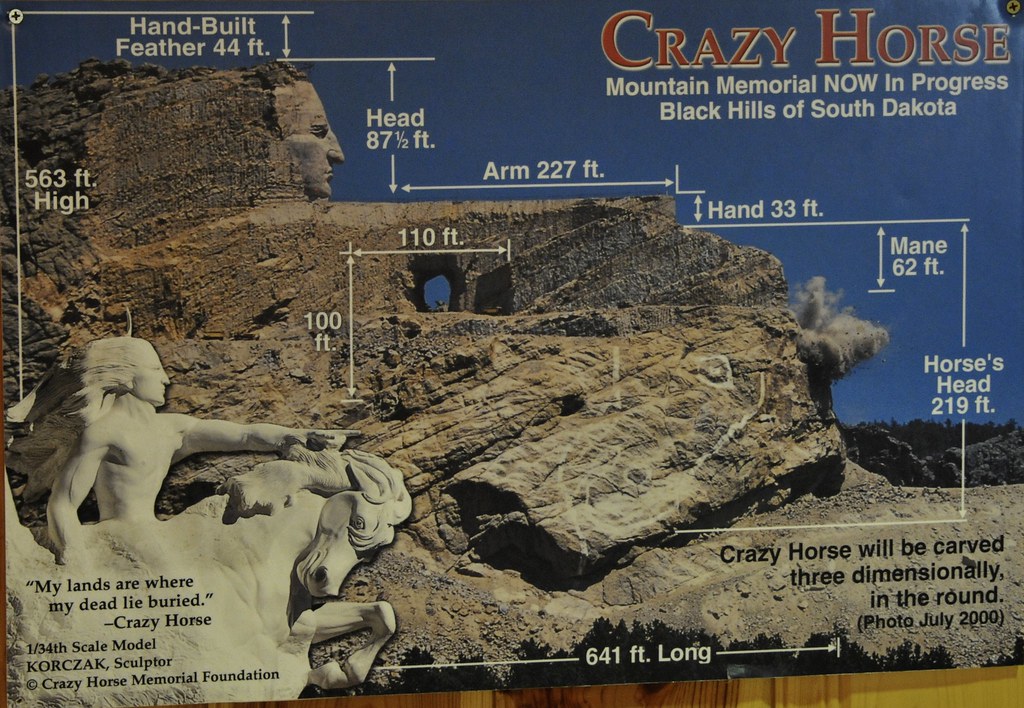The image showcases an informational board about the Crazy Horse Mountain Memorial in progress in the Black Hills of South Dakota. The centerpiece of the photograph is a mountainside with partially carved sections and various measurement lines indicating the ongoing progress. In the top right, red and white text announces "Crazy Horse Mountain Memorial now in progress Black Hills of South Dakota." The bottom right of the board reads, "Crazy Horse will be carved three-dimensionally in the round. Photo July 2000." The bottom left displays a completed concept illustration of a man riding a horse, labeled with black text: "My lands are where my dead lie buried - Crazy Horse. 1/34th scale model. Korczak, sculptor. Crazy Horse Memorial Foundation." The entire scene is mounted on a wooden wall, giving context to the ambitious scale and intricate details of the monumental project.